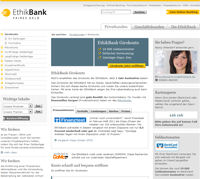In the upper left corner of the image, there is a yellow circle. Next to this circle, in black text, is the word "ETHIK," followed by the word "Bank" in a slightly darker black font. On the right side of the image, there is a yellow banner with black text inside, but the text is small and blurry, making it difficult to read.

In the center of the image, there are two dark green rectangular boxes. One of these boxes contains white text, and below it, there is another yellow banner with some additional text inside. On the right side of the person with dark brown hair, a woman is pictured. She is smiling, with text both above and below her photo, though the text is very small and blurry.

Towards the bottom center of the image, there is a blue rectangle containing white text. Additionally, there is a search bar located at the top of the image, near the Ethik Bank logo, with a few letters typed into it. Next to the search bar, there is a small gray rectangle with the word "SEARCH" inside.